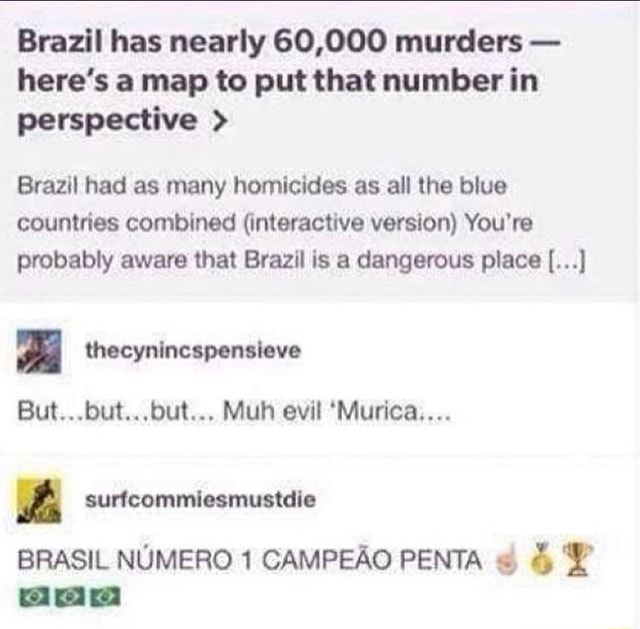The cropped screenshot appears to be a potential meme, featuring a news headline in bold black text: "Brazil has nearly 60,000 murders. Here's a map to put that number in perspective." There is an arrow pointing towards where the map would presumably appear, but the map itself is not visible. The smaller text below reads: "Brazil had as many homicides as all the blue countries combined. Interactive version. You're probably aware that Brazil is a dangerous place and..." with an ellipsis indicating the continuation of the story.

Beneath the main text, there are two user comments. The first comment, made by a user named "The Sinning Spin Sieve," sarcastically states: "But, but, but my America, my evil America." The second comment, from a user named "Surf Commies Must Die," declares: "Brazil numero uno, Campea Penta," followed by emojis including a hand making a number one sign, a number one medal, a trophy, and three Brazilian flags.